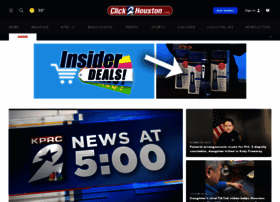The image depicts a small, low-resolution screenshot of a website viewed on a computer. The top portion of the image features three horizontal bars aligned consecutively. The uppermost bar is black and includes an indistinct red and white icon in the center, likely representing the website's logo. Beneath this, a second, muted black bar displays nine white words, which appear to be navigational buttons or links, though the text is illegible. The third bar below is green with blurred white text that is also unclear.

Continuing down the image, there is a larger horizontal photograph depicting a group of people gathered indoors, potentially at a concert. Many participants appear to be holding candles, suggesting a vigil. The image caption, although blurry, seems to read something similar to "Forever 12, Family Holds Candlelight Vigil" followed by three indistinct words and then "Friday morning".

To the right side of this photo is a small section seemingly dedicated to the weather forecast, displaying data for three days, likely intended for user interaction. Below this section is another area with more white blurry text and an image of two men standing near a car, though further details are hard to make out.